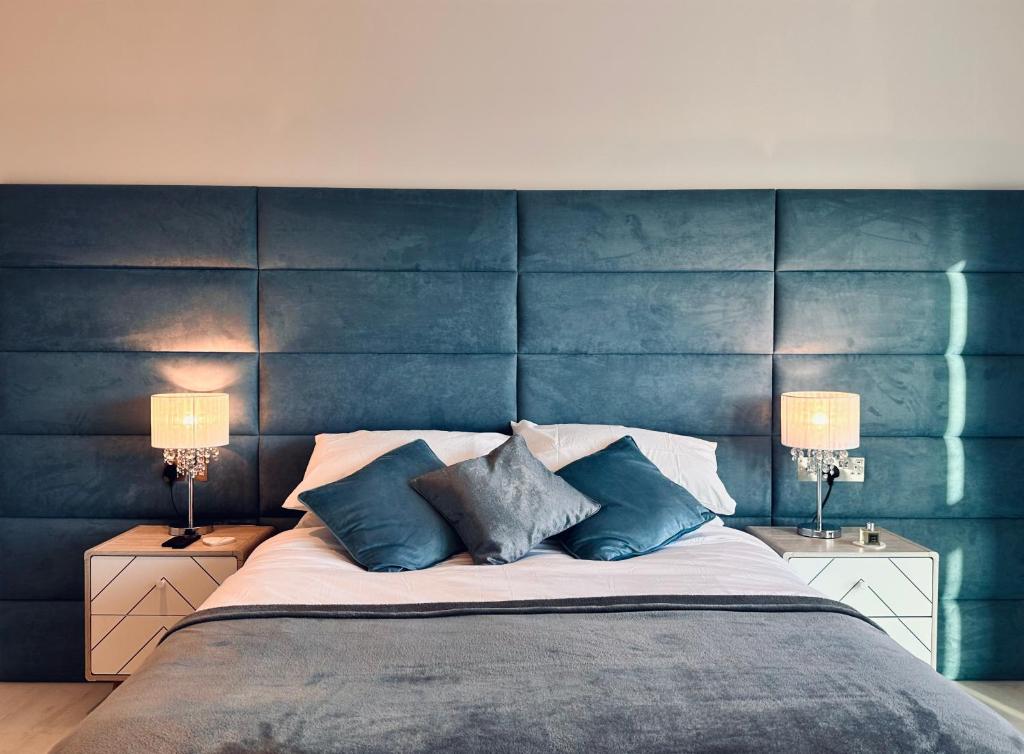This photograph captures a stylish bedroom, featuring a queen-size bed with a gray, velvet-like comforter folded down to reveal a white interior. The bed is adorned with white pillows and three decorative throw pillows—two in blue and one in gray. The backdrop to the bed is a striking, blue, textured headboard composed of large rectangular panels that span the entire width of the image. Above this headboard, the wall is a contrasting cream color. On either side of the bed are nightstands, each hosting a lamp with a silver base, white lampshade, and delicate chandelier-like hangings. The nightstands, adorned with a few indistinct items, complement the room's cohesive color palette and design aesthetic.